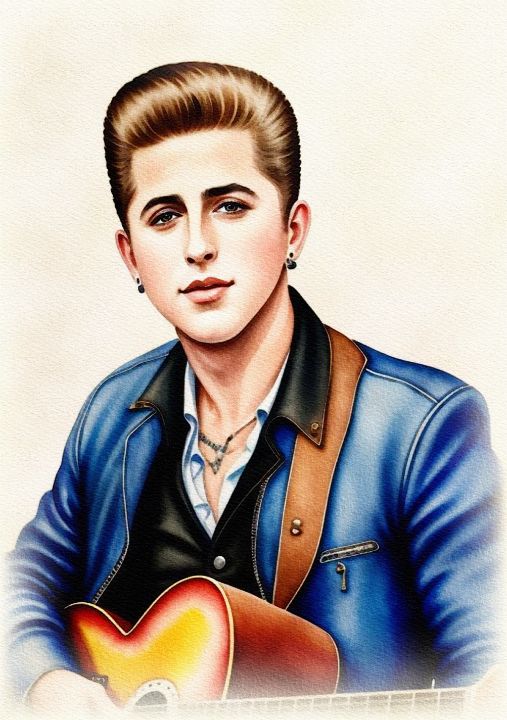In this image, a man with slicked-back brown hair and sideburns is depicted holding a guitar. He is dressed in a blue suit with a black vest that has a collar, and beneath it, he wears a blue button-down shirt layered over a white collar shirt. The man, who bears a resemblance to a blend of Elvis and Brandi Carlile, is smiling and looking straight ahead. His accessories include earrings in both ears and a beaded necklace around his neck. One notable detail of his attire is a zipper on the left side of his chest. His guitar, featuring a brown body with orange and white accents, is supported by a brown strap and is being strummed by his right hand. The portrait captures him from the top of his head to just above the waist, showcasing a glimpse of his left arm down to the elbow and a larger portion of his right arm. The background of the picture is primarily pink around his head and shoulders, fading to white towards the bottom corners, further emphasizing the subject's features.